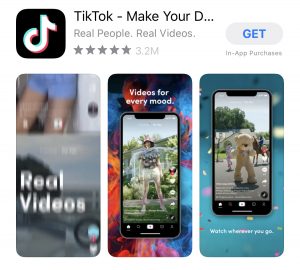This image is an advertisement for TikTok. At the top, a black square features a white music note icon outlined in blue and pink. To the right of the icon, bold text reads "TikTok - Make Your..." followed by three dots. Beneath this slogan, it states "Real people. Real videos," and highlights a rating of five stars from 3.2 million downloads. 

Directly below, there is a rectangular button that displays the word "GET" in capital letters, indicating an option to download the app.

Under the download button, there are three images of cell phones, each showcasing different aspects of TikTok:

1. The first phone showcases "Real Videos."
2. The second phone displays "Videos for Every Mood" and features an image of a woman standing in a garden, wearing shorts, a short-sleeved shirt, and a hat.
3. The last phone image shows a person dressed in a teddy bear suit with people dancing behind them on the road. The accompanying text reads "Watch Wherever You Go."

The background of the advertisement is a vibrant blue with pink and white dots scattered throughout.